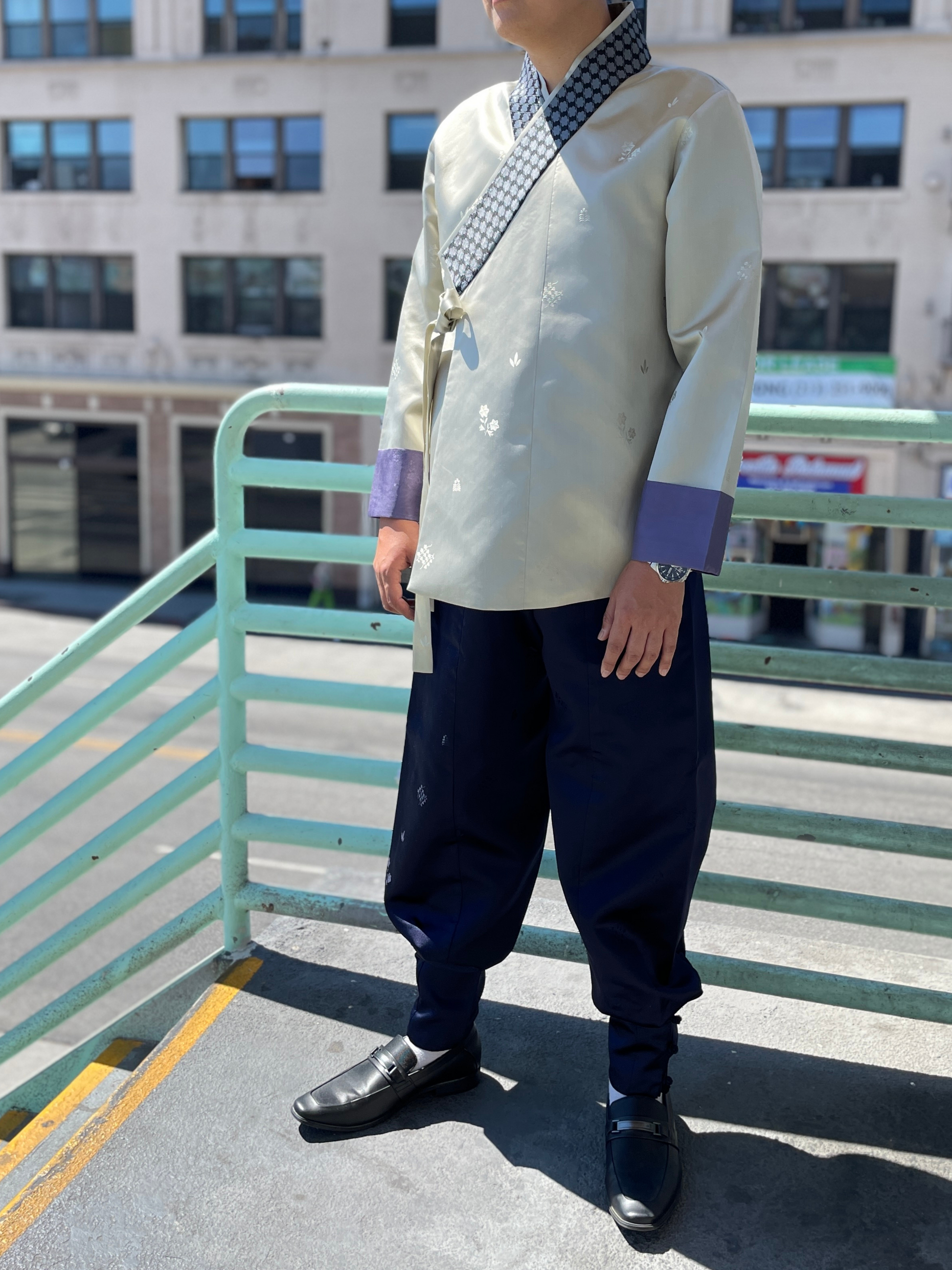In the image, a man of Asian descent stands at the top of a cement staircase with yellow paint on the edges of each step. Behind him is a seafoam green metal railing. The outdoor setting features an industrial cityscape, including a building with numerous windows that appear to be either apartments or commercial spaces, and a sign in blue and red that cannot be clearly discerned.

The man showcases a traditional Asian outfit. His top is white with a blue and gray patterned collar that folds over, and it is detailed with purple cuffs at the tips of the sleeves. The top wraps around and ties at the side, reminiscent of martial arts attire. He sports a silver watch on his left wrist. His black pants are baggy, ending just above his ankles, and he wears black leather loafers paired with white socks. His stance is upright, exuding confidence as he presents his ensemble.